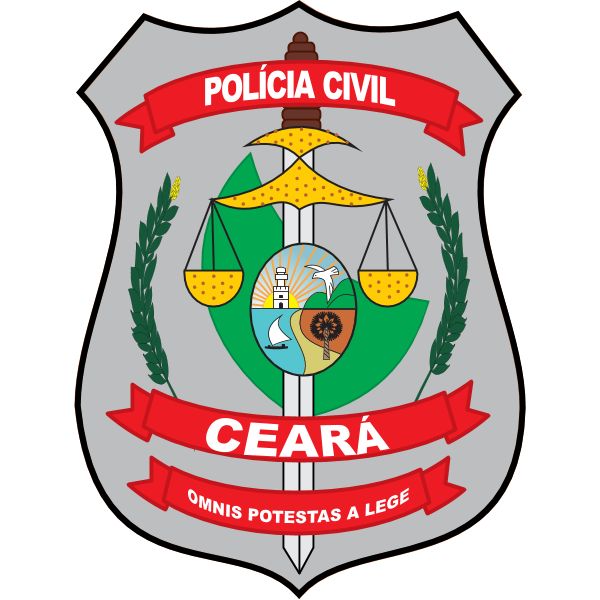This image displays a computer-generated police badge with a black outline and a solid medium gray background. At the top of the badge, a red banner with white lettering reads "Policia Civil." Central to the badge is an intricate design featuring a downward-facing sword, with the scales of justice integrated into the sword's handle. The scales have a yellow background with small brown dots and consist of a triangle shape with a curved bottom, and hanging semi-circles with lines attached. Surrounding this central imagery is an oval containing detailed illustrations: a lighthouse, a white dove flying leftward, a windmill, a tree, and a sailboat. Beneath this, at the lower part of the badge, another red banner reads "Ceara," and a final red banner at the very bottom displays the phrase "Omnis Potestas a Lege." Flanking the scales of justice are two green fern leaves, adding further detail to the badge's sophisticated design.